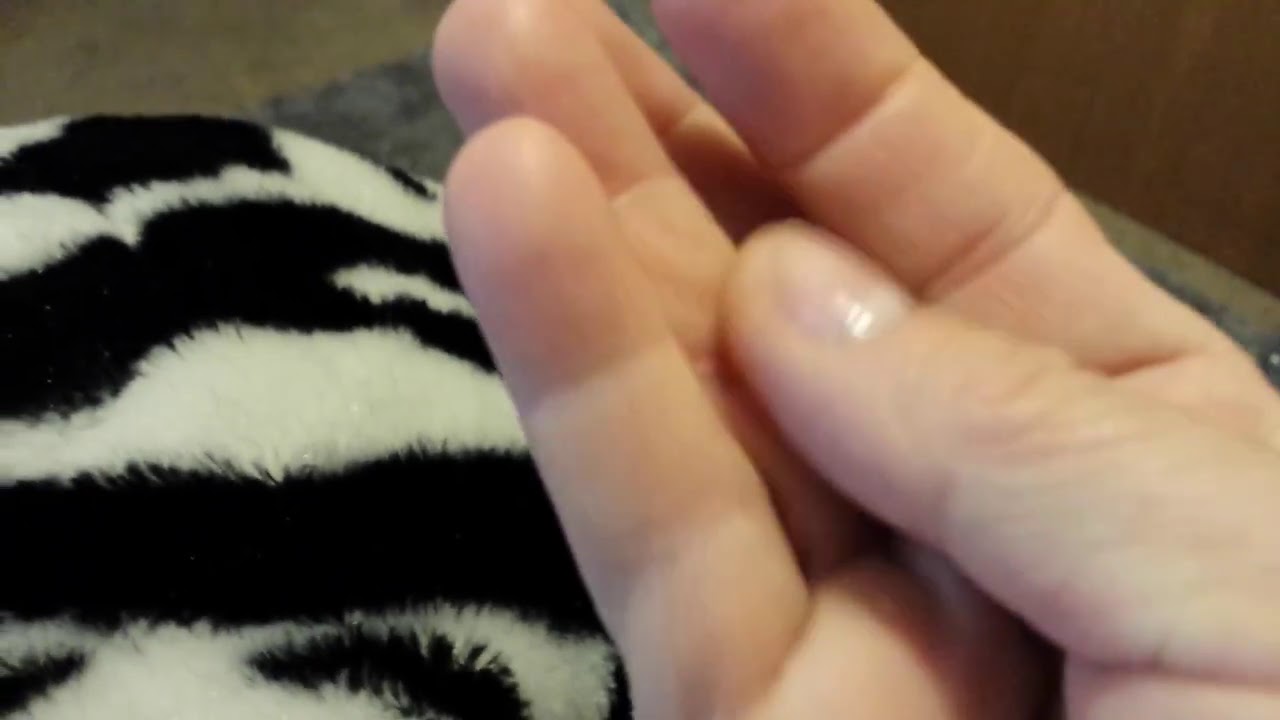This close-up photograph showcases a clean and well-groomed right hand, positioned predominantly in the bottom right of the image. Viewed from the palm side, the thumb is folded over and touching the middle two of the four clearly defined fingers, which are slightly pinched together. The nails are trimmed neatly, with the thumbnail distinctly visible. The background reveals a black and white zebra-patterned blanket draped over what appears to be someone's legs. At the top edge of the image, there is a glimpse of grayish-bluish carpeting. Additional details include a brown wooden object near the top right and a subtle indication of tile flooring underneath. The hand, seemingly belonging to a Caucasian individual, does not hold any objects.